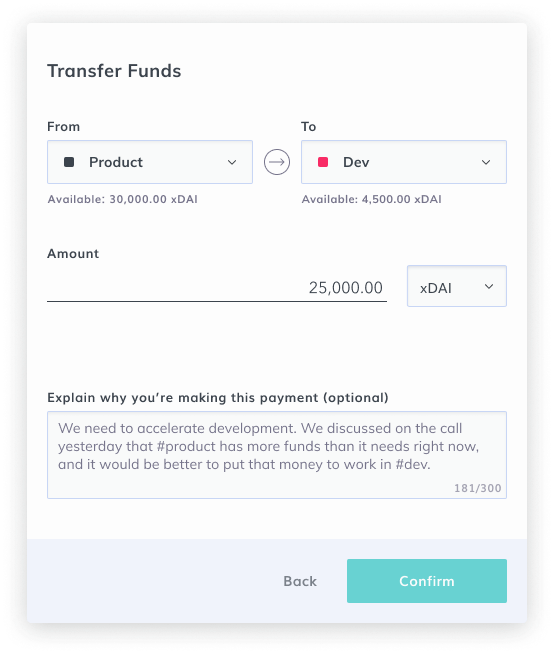The image depicts a detailed transfer funds interface with a primarily white background featuring both black and gray text and subtle color accents on certain icons and buttons. At the top, the section is titled "Transfer Funds". Below this, there are clearly labeled "From" and "To" sections. 

The "From" section is labeled "Product" and is accompanied by a black square. The "To" section is labeled "Dev" with a red square next to it. Under each section, there is text indicating available funds; the "Product" side displays "Available $30,000 XDAI", and the "Dev" side shows "Available $4,500 XDAI".

Below these sections is an "Amount" field populated with "$25,000", and a dropdown next to it indicating the currency "XDAI". Further down, there's an explanatory text box prompting the user to explain the reason for the transfer, marked as optional. Inside the text box, the pre-filled message reads: "We need to accelerate development. We discussed on the call yesterday that #Product has more funds than it needs right now, and it would be better to put that money to work in #Dev", with a character count displayed as "181/300".

At the bottom of the image, there is a back button and a prominent turquoise button with white text that says "Confirm", which users can click to finalize the fund transfer. This interface provides a straightforward and intuitive way to manage fund allocation between different sections while ensuring transparency and clarity in the transfer purpose.